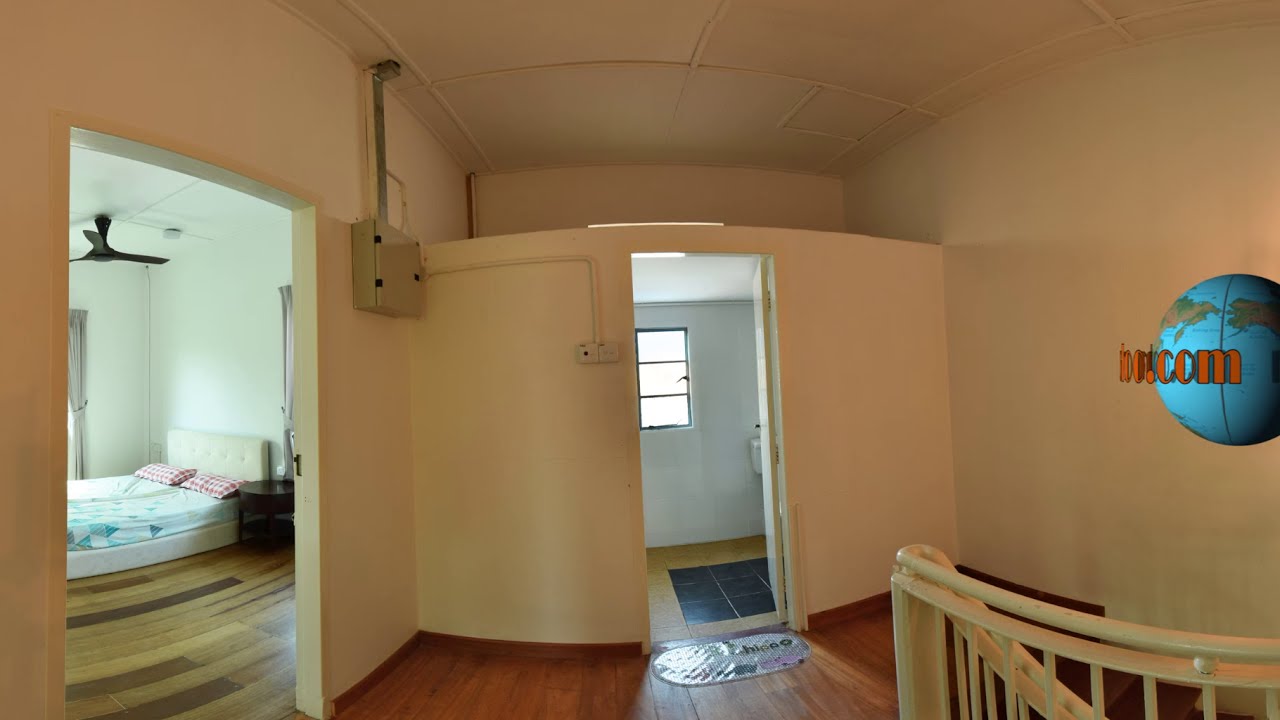The image captures the interior of an upper floor in a home, presenting a detailed view of a central hallway. The ceiling is off-white with various seams visible. Dominating the middle of the image is an open door leading to a bathroom, revealing a black tile floor that contrasts with the surrounding tan wooden floor. A dark brown wooden floor extends in front of the bathroom door, and an off-white staircase railing made of metal ascends to meet the landing area. On the right side, just outside the bathroom, an electrical fuse box is mounted on the wall.

To the left of the central hallway, another open door leads into a bedroom. This room features a king-size bed with a tan fabric headboard and designer blue bedsheets complemented by red and white checkered pillowcases. A black ceiling fan is visible above the bed, and the bedroom includes an end table and a window with open curtains, allowing light to flood the space. The walls throughout are painted off-white, contributing to a clean, bright atmosphere. The flooring continues with a wooden design that complements the home's overall aesthetic. In front of the bathroom door, a doormat is visible, adding a touch of homeliness to the scene.